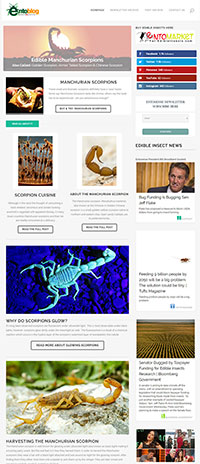This is an edited screenshot of the homepage of the "Into" blog designed for mobile landscape view. The layout features a white background and visually scattered thumbnails of scorpions. The "Into" blog logo appears prominently in the top left corner. Adjacent to this logo is a large photo of a scorpion overlaid with white text. On the right side of this logo is the "Into" logo repeated. To the right of the large scorpion image is a vertical list of social media accounts represented in rectangular bars. Below the social media links, there is an advertisement presented as a white box with blue text and a button at the bottom. The page is notably long, and instead of a scrollable interface, the content appears laid out in its entirety within a single image.